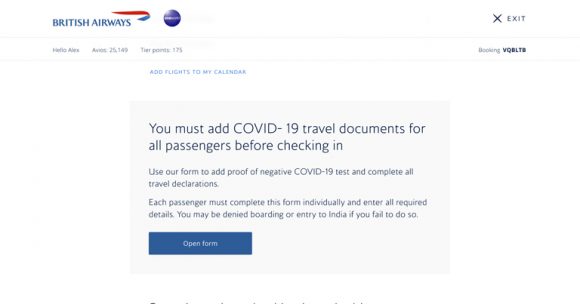At the top left of the image, "BRITISH AIRWAYS" is prominently displayed in all capital letters using a dark blue font. Towards the upper right, there is a ribbon that transitions from red at the top to blue towards its tip, which points to the right. Adjacent to this ribbon, a spherical shape in a purplish-blue hue appears, featuring some white text at its center that is too small to decipher.

Further to the right, there is a black "X" symbol followed by the word "EXIT" in black, capital letters with significant spacing between each letter. This section is followed by a light gray divider.

Below the divider is a menu area. The menu begins with the text "Hello, Alex" in small black font. The subsequent section is partially unclear, but it includes "Tier Points: 175." Below this, in blue capital letters, it reads "ADD FLIGHTS TO MY CALENDAR."

Continuing downward, there is a rectangular section with a light gray background. At the top of this section, large dark bluish text states, "You must add COVID-19 travel documents for all passengers before checking in." Below this, smaller text reads, "Use our form to add proof of negative COVID-19 test and complete all travel declarations. Each passenger must complete this form individually and enter all required details. You may be denied boarding or entry to India if you fail to do so."

Towards the bottom left of this section, there is a rectangular dark blue icon. In its center, thin white lettering reads, "OPEN FORM."